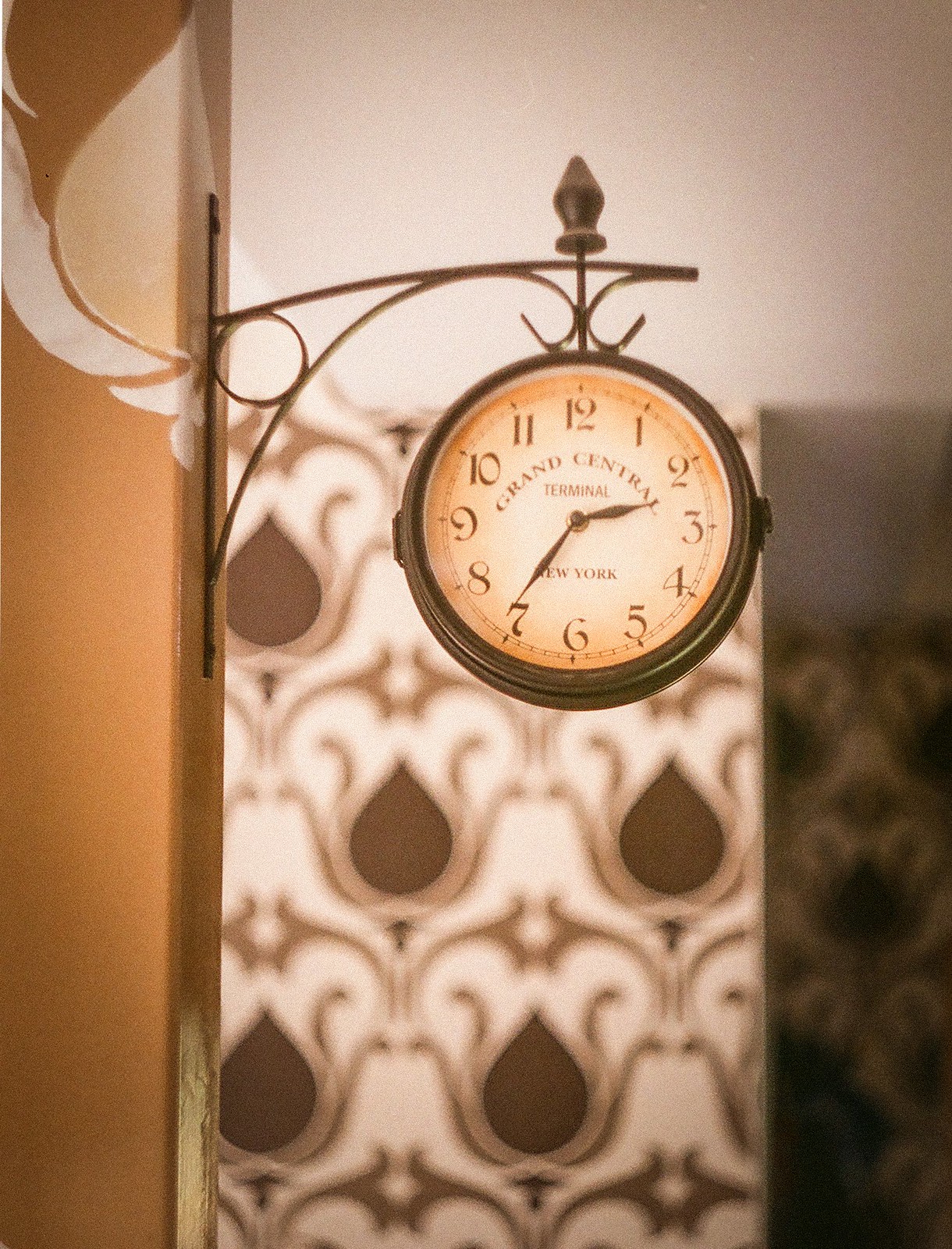The image captures an ornate corner of a building featuring a blend of traditional and decorative elements. On the left side, there's an orangey-tan wall. Attached to this wall, a long black metal strip, likely cast iron, extends vertically. From this strip, a wrought iron arm stretches out to the center of the image, showcasing intricate curved and circular designs. Suspended from this ornate arm is a prominently placed clock. The clock has a brown outline and an aged, yellowed tan face. It prominently displays the words "Grand Central Terminal, New York" at its center, surrounded by traditional numbers marking 12, 3, 6, and 9 o'clock positions. The clock reads approximately 2:37. The background features an ornate, Persian or Moroccan-style wallpaper in cream, tan, and dark brown, adorned with intricate teardrop shapes and patterns. The overall composition creates a visually rich and culturally infused scene.